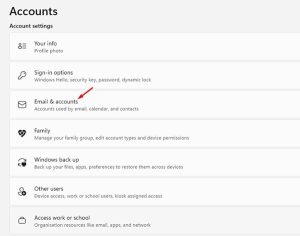The image displays a webpage section dedicated to account management, presented with a gray background. At the top, the title "Accounts" is prominently displayed in bold black lettering. Directly below, in significantly smaller text, the header reads "Account Settings."

The content is organized into distinct white boxes that span the width of the page, each containing different account management options. Starting from the top, the first box is labeled "Your Info," followed by "Sign In Options" in the second box. Though somewhat challenging to read due to the small font, a brief description accompanies each label.

The third section, marked "Email and Accounts," features a red arrow pointing downward towards the "Accounts" title, adding a visual cue. Next is the "Family" section, which is distinguished by an adjacent heart icon. Another section is labeled "Windows Backup," which is followed by a section that appears to be labeled "Other Users," though it's slightly unclear. The final section is titled "Access Work or School."

The illustration offers no specific information on the website or company the page belongs to. It appears to be a segment of a larger site, presumably one where previous instructions or information was provided, and this is the subsequent section users encounter. The layout is user-friendly, with each category neatly compartmentalized in individual white boxes that extend from the left margin to the right, ensuring clarity and ease of navigation.